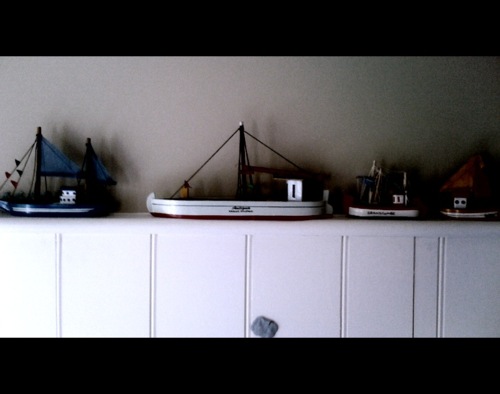This photograph, taken indoors with ambient low light, captures a horizontally broader scene than it is tall. At the immediate top and bottom are black letterboxes framing the image. Below the top letterbox, a flat-screen TV edge is subtly visible. The main focus is a white cupboard, about 40-45% of the image at the bottom center, against a light brown, tan wall. The cupboard features three vertical closed cabinets. Atop the cupboard, four model boats are laid out from left to right.

The first boat on the left is a dark blue model with several blue sails. Next to it is the largest ship, white with a prominent red underside, equipped with a mast but no visible sails. The third and fourth boats are progressively smaller, making them harder to discern under the shadowed lighting conditions. The third boat, appearing like a tugboat, is white with black accents. The final boat on the right is a smaller vessel featuring a red sail and a white body with more red accents. The overall atmosphere suggests it might be late afternoon or an indoor setting with minimal lighting, casting shadows that obscure finer details of the model boats.